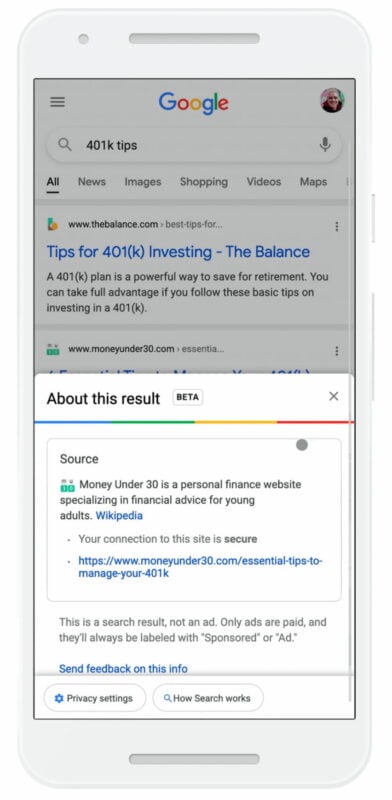This image is a detailed screenshot of a cell phone displaying a Google search results page. 

The phone is visually outlined by a light blue border, about one inch thick on the top and half an inch on both sides and the bottom. At the very bottom center of the phone, slightly upwards from the edge, there is a dark gray area that houses a speaker. A similar dark gray area is at the top, also containing a small circle to the left of the speaker. The screen is framed by a black border.

The upper half of the screen is slightly shaded to indicate a pop-up tab. The white bottom half of the screen displays the main search results. At the top center of the screen, the word "Google" is displayed. On the top right, there is an icon profile of a man, and on the top left, there are three black horizontal lines representing the menu.

Below the Google logo is a search bar with the text "401k tips" in black. Underneath the search bar are tabs labeled "All" (bolded and underlined), "News," "Images," "Shopping," "Videos," and "Maps," all in black. 

The first search result is shown as follows:
- A site icon is to the left with the URL "www.thebalance.com."
- The clickable title "Tips for 401k Investing - The Balance" in blue.
- Three lines of black text summarizing the content.

The pop-up tab at the top left says "About this result" in bold black text, alongside a small white tab marked "beta" in black. An 'X' icon is situated on the right side for closing the pop-up.

Below this, a line segmented into four colors: blue, green, yellow, and red, represents Google's branding. Following this line, there is a gray-outlined square with "Source" in the top left corner, accompanied by textual information spread across two lines. Next to it, Wikipedia is marked in blue, followed by a black line and a clickable link beneath it. Below, two lines of additional information are presented, with another blue clickable portion for more feedback.

On the left side of the pop-up tab, there is a white section with a blue settings icon reading "Privacy settings." On the right, another white section says "How search works" in black.

This comprehensive layout provides clear insight into the search results as viewed on a mobile device.